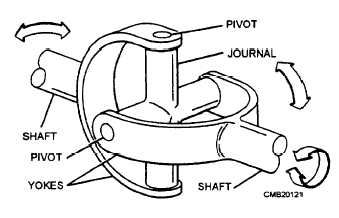This small, horizontal image is an exploded drawing of a piece of equipment. It features no border and centralizes on components joined together, with additional parts labeled externally. At the heart of the drawing is a vertical cylinder crossing a horizontal cylinder, forming an X-shape. Attached to this intersection are two metal pieces resembling spurs; one is mounted vertically on the vertical cylinder. Various labels indicate components such as "pivot," "journal," "shaft," and "yokes." There are arrows in the image depicting rotational directions, including a circular arrow and two others pointing left and right, which illustrate the motion of each part of the universal joint. The text "CMB2012H" appears below the last arrow, located at the bottom right-hand corner of the image.